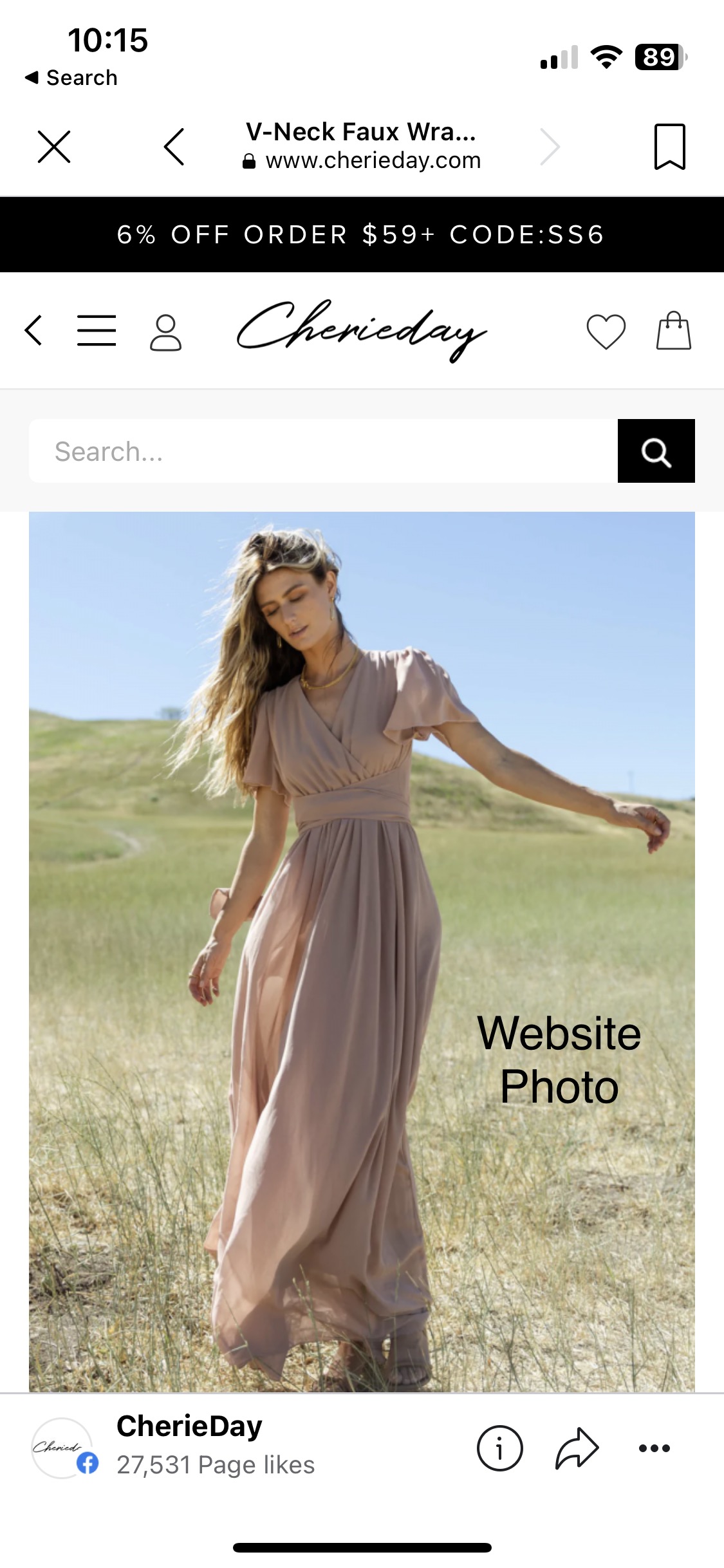The image features a predominantly black bar at the bottom and a detailed top section displaying various elements: the time '10:15', a search button on the left, signal strength showing 2 to 4 bars, full wifi signal icon, an 89% battery indicator, and several text elements including 'X', 'VNIC', 'fall', 'rad', and the website 'www.sherryday.com'. Additionally, there is a promotional banner indicating '6% off $459 plus code SS6'. A left arrow is also visible along with several dashes.

In the center of the image, there is a clear and significant focal point: Sherry Day, a person whose name is highlighted with a heart icon beside it. She is depicted standing on a grassy hill under a blue sky with dirt hills and grass surrounding her. She is wearing a wavy pink dress, adding a striking contrast to the natural backdrop.

Further details include a magnifying glass symbol indicating a search function, blue lines to the right of the main image labeling it as a 'website photo', and 'Sherry Day 27,531 page likes' placed at the bottom left corner. There is also a circular icon with an 'i' in it and a dot arrow pointing to the right, followed by an ellipsis ('...') suggesting additional options or information.

Overall, the image weaves together elements of a webpage interface and a serene landscape scene with Sherry Day centrally positioned, blending technology with nature.